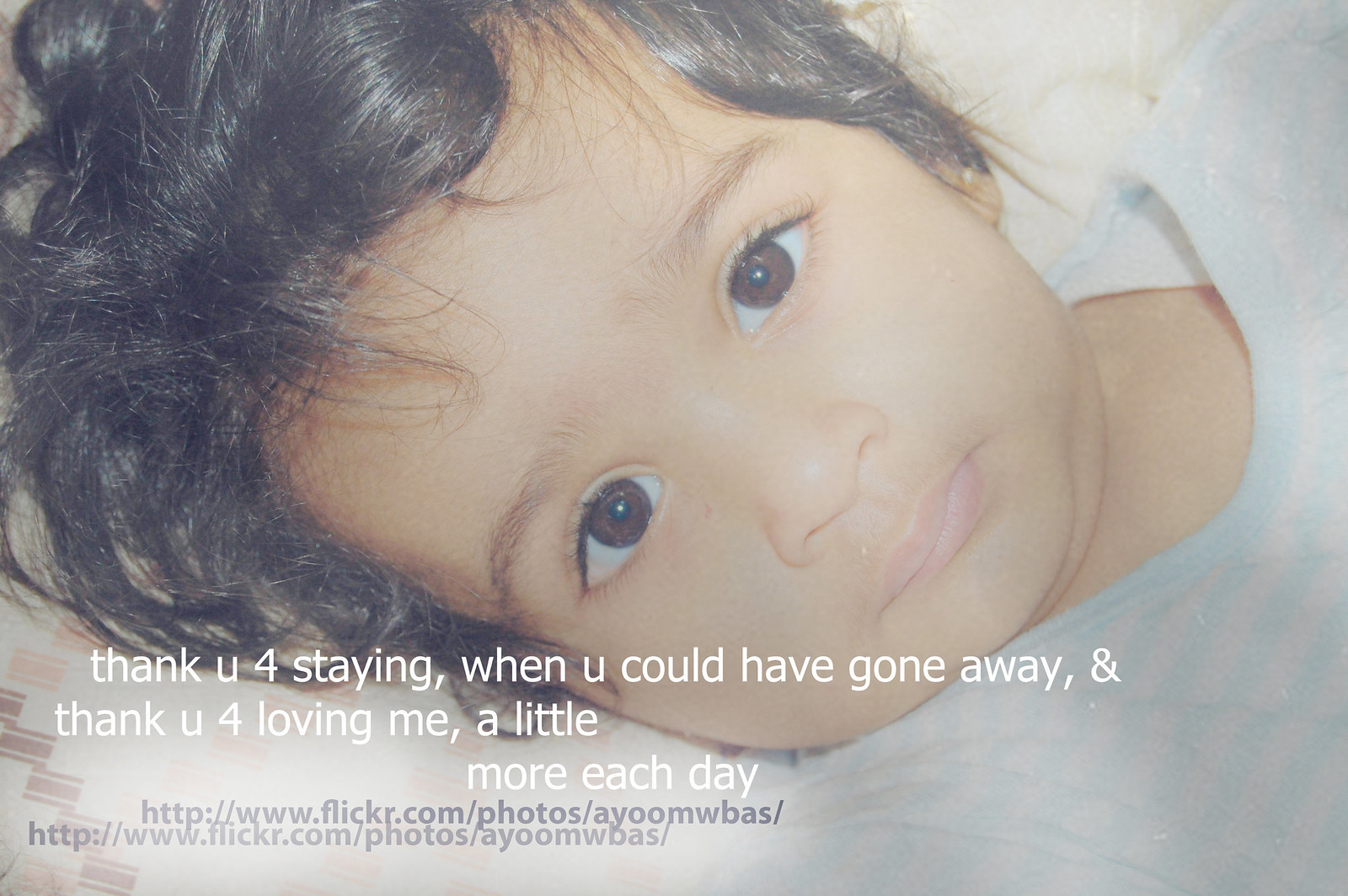This full-color photograph captures a young baby, likely around a year old, lying on her right side with her head taking up most of the frame and positioned to the left. Her dark, curly hair is tousled, suggesting she may have been sleeping. She has wide, brown eyes staring directly at the camera with an expressionless face. The baby is dressed in a white top. Text in white at the bottom left of the image reads, "Thank U 4 staying when you could have gone away, and thank you for loving me a little more each day." The text uses the numeral "4" for "for" and the letter "U" for "you." There are also watermark URLs at the bottom in dark lettering indicating the photographer's website, "http://www.flickr.com/photos/AUMWBAS." This photograph could be interpreted as a promotional piece from an anti-abortion group, given the context of the message.